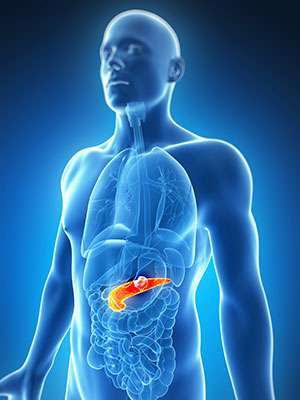This image is a highly detailed, blue-tinted illustration of a man's body that resembles an x-ray. The man's body outline is highlighted with a light blue line, and it features a bald head with closed eyes and glowing lips. The illustration provides a translucent view of internal organs, showing the esophagus descending into the lungs, intestines with visible ripples, and the stomach. Notably, a peculiar organ is depicted just above the large intestine; this organ is brightly lit in orange and yellow, shaped somewhat like a tilted letter 'J' or half of a boomerang, with sharp points at the top and a rounded bottom. A white, ball-like substance is visible within this orange organ, making it stand out even more. The background of the image transitions from a dark black at the top corners to a light blue hue towards the center, enhancing the luminous and artificial aesthetic of the illustration.